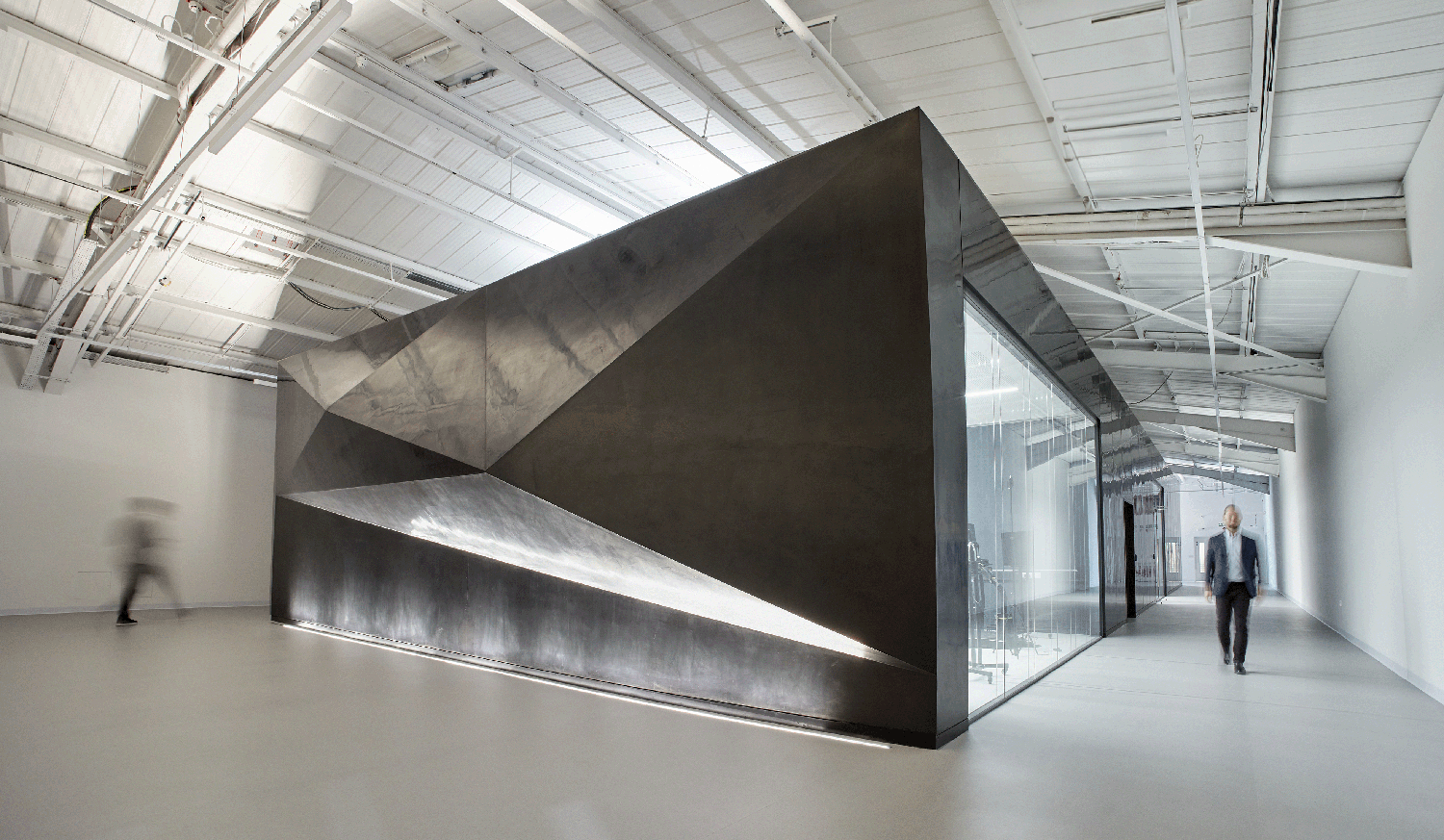The photograph depicts an expansive, sleek warehouse or factory space with white-painted walls, high vaulted ceilings, and a polished white floor. The ceiling architecture includes visible pipes and metal beams, contributing to an industrial yet modern aesthetic. Dominating the center of this cavernous space is a striking rectangular structure with a black, metallic sheen and a glass front wall that hints at an interior working or gallery space. The structure also features geometric designs and angular shapes along its sides. 

To the right of this central unit, a man in a black coat, white shirt, and black pants walks toward the camera. White walls accompany him on his right as he traverses what appears to be a hallway. On the far left, another man can be seen in motion behind the black structure, although he appears blurry due to the movement captured during the shot. The image balances the contrast between the bright, open warehouse area and the sleek, dark central structure, enhancing the sense of space and modern functionality.